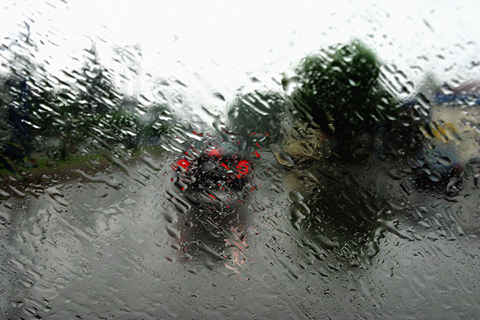The image depicts a blurred view through the rain-streaked windshield of a car. The scene outside is obscured by water droplets, creating a hazy appearance. Through the blur, a road is visible with a car directly ahead; its red taillights and third brake light glowing distinctly through the rain. The sky is overcast with a light blue hue, and the wet pavement below appears gray. To the sides, there are vague outlines of trees, with some green hues on the right and possibly another vehicle or object further to the right. The overall setting suggests a rainy drive with diffuse, muted colors dominated by the gray road, cloudy sky, and the red lights of the car in front.